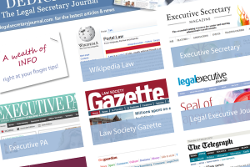This image showcases a website featuring an extensive directory of British newspapers and journals, arranged in a visually organized yet angled layout. The topmost entry, although partially obscured and abbreviated as "D.E.D.," is linked to Marissa Lesikoff and titled "The Legal Secretary Journal." Below this, another entry reads "A Wealth of Info, right at your fingertips."

Further down, the list includes "Wikipedia" associated with "Wikipedia Law," characterized by straightforward labels. Following this, "Executive Secretary Magazine" is presented with a considerable amount of tiny, unreadable text, underlined by a blue banner labeled simply "Executive Secretary."

To the left, we have "Executive P.A." marked by white text on a blue buttoned banner. Below this, the "Law Society Gazette" stands out with its maroon background and white lettering, supplemented by a clickable blue button. Next, the "Legal Executive" is mentioned, accompanied by a blue button labeled "Legal Executive Journal."

The leftmost entry is partially cut off, revealing only the top of a maroon banner. Adjacent to it, in the middle of the screen, a portion of "The Guardian" can be seen, although its headings remain indecipherable. Finally, "The Telegraph" appears at the bottom right, complete with selectable menu options rendered in a mix of black and blue text.